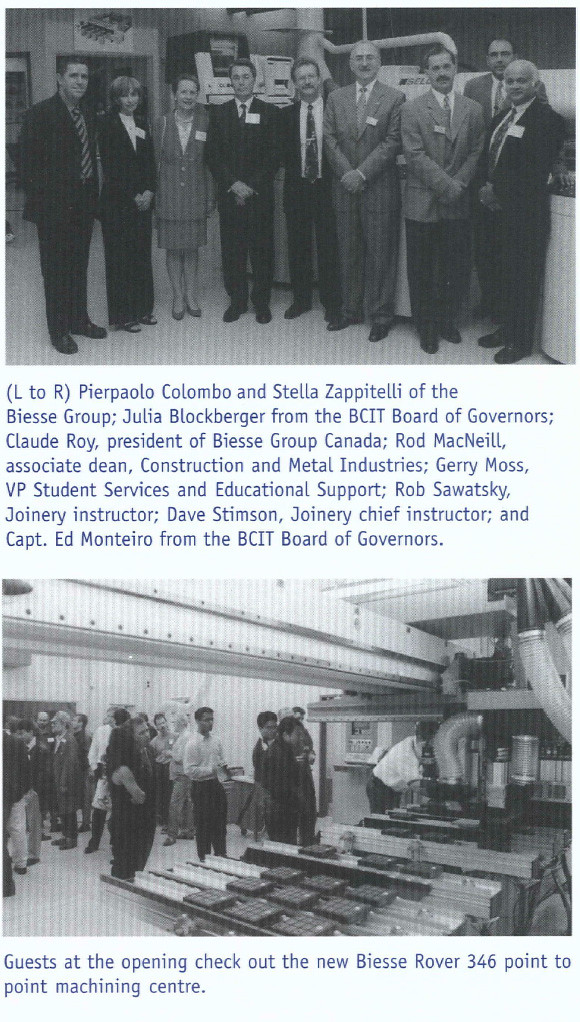This vertically aligned rectangular image, resembling a page from a magazine or newspaper, showcases two black-and-white photographs, each with detailed captions underneath. The top photograph features a formally dressed group of approximately ten individuals, including mostly men with a few women. They are dressed in business suits, ties, and professional attire, standing in a formal lineup. The caption below this photo, aligned to the left against a potentially light blue or white background, lists their names and roles, identifying them as members of the BSE Group, including the Board of Governors and various officials from construction, metal industries, and educational support sectors.

Beneath this is another black-and-white photograph depicting a different group of individuals amidst a facility tour, surrounded by machinery. The caption under this image reads, "Guests at the opening check out the new BS Rover 346 point-to-point machining center," indicating that the group is inspecting technological advancements within the facility. The overall setting suggests a formal event and provides a historical snapshot of a significant corporate and industrial occasion.